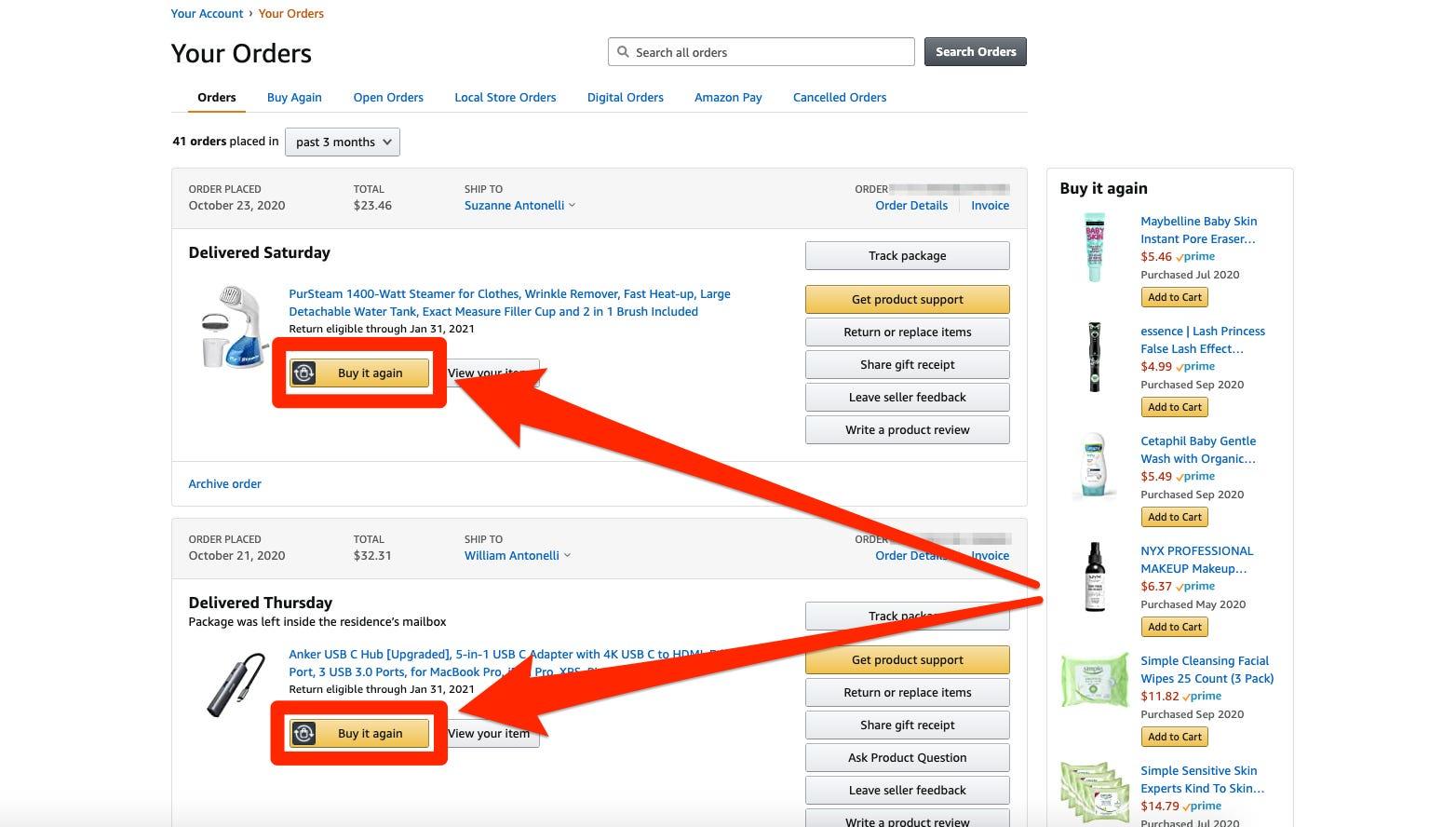The image displays a screenshot of the Amazon website, specifically focusing on the "Your Orders" page. At the top, the "Your Account" section is highlighted in blue, while the "Your Orders" section is marked in a prominent orange color. The "Your Orders" heading is bolded in black.

A search bar with a magnifying glass icon is positioned at the top, enabling users to search through their orders. Below the search bar, several order-related options are listed in blue hyperlinks: "Buy Again," "Open Orders," "Local Store Orders," "Digital Orders," "Amazon Pay," and "Canceled Orders." The page indicates that 41 orders have been placed in the past three months, with a dropdown menu available to adjust the time frame.

One specific order is displayed, placed on October 23rd, 2020, totaling $23.46 and shipped to Suzanne Antonelli. This order, marked as delivered on a Saturday, includes a red arrow pointing to the "Buy Again" option, highlighting a Pure Steam Steamer for Clothes. Users have various options for this order, such as tracking the package, getting product support, returning or replacing items, sharing a gift receipt, leaving seller feedback, or writing a product review.

Another item listed is a USB adapter, delivered on a Thursday for $32.31 to William Antonelli. Similar to the previous order, there are "Buy It Again" options available on the right side of the screen.